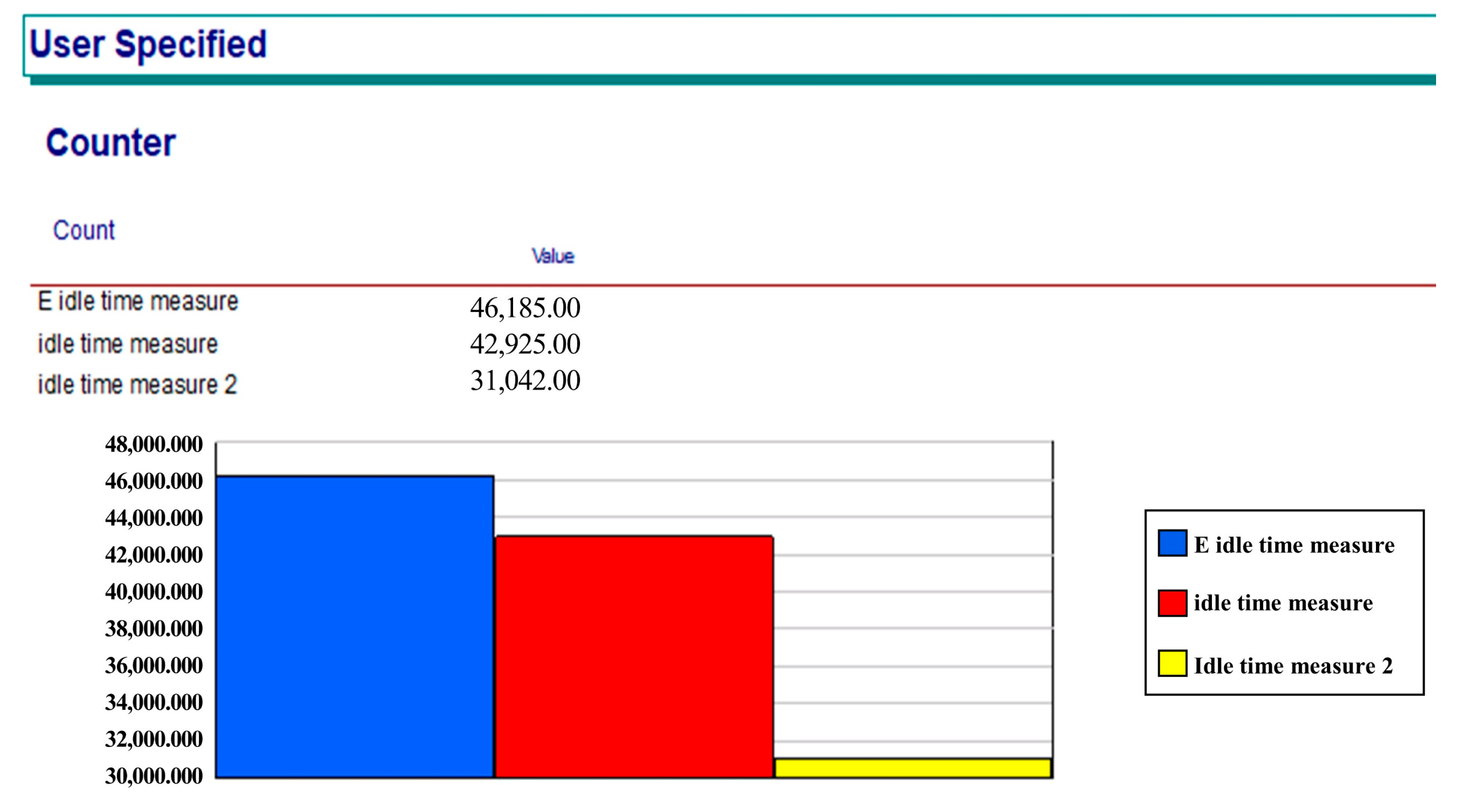The image displays a chart with a white background and no formal border. At the top left corner, "user specified" is written in blue font, followed by a teal-colored horizontal line. Below this, another blue text reads "counter," underneath which are two columns labeled "count" on the left and "value" on the right. The table comprises three rows: the first row lists "E Idle Time Measure" with a value of 46,185, the second row shows "Idle Time Measure" with a value of 42,925, and the third row indicates "Idle Time Measure 2" with a value of 31,042.

To the left of the table is a bar graph that visually represents these values. The graph features three bars on the x-axis: a large blue bar for "E Idle Time Measure," a shorter red bar for "Idle Time Measure," and a very thin, low yellow bar for "Idle Time Measure 2." The y-axis includes numerical increments ranging from 30,000 to 48,000.

Situated to the bottom right of the image is a key explaining the color-coding: blue corresponds to "E Idle Time Measure," red denotes "Idle Time Measure," and yellow represents "Idle Time Measure 2." The visual and numerical data provide a clear comparison of the three measures, indicating that "E Idle Time Measure" has the highest value, followed by "Idle Time Measure," and "Idle Time Measure 2" has the lowest value.